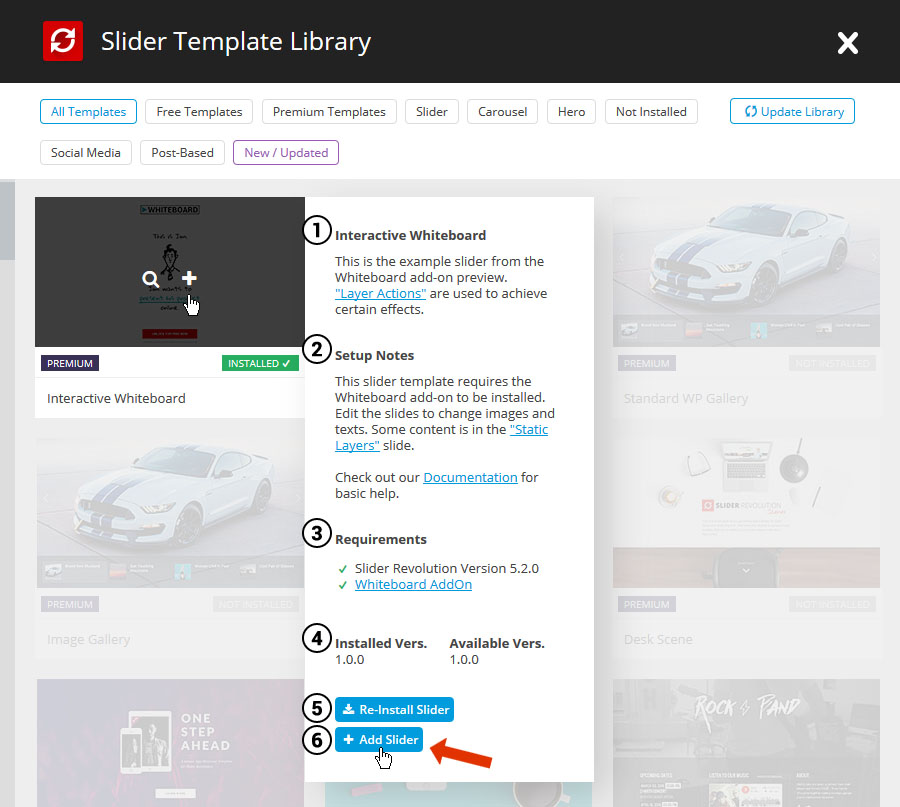The website interface features a prominent black bar at the top, which contains a slider and a template library. To the left of the bar is a red box, and to the right, circular icons with two arrows and an 'X' button are displayed. The bar is followed by text that lists various template categories: "All Templates," "Free Templates," "Premium Templates," "Slider," "Carousel," "Hero," "Not Installed," and a blue "Update Library" button.

Beneath this section, there are tabs labeled "Social Media," "Post Based," and "New/Updated," each highlighted in a purple box with purple lettering. Below these tabs, there is a vertically oriented black box containing a question and a plus sign, labeled "Interactive Whiteboard." An example slider from the whiteboard demonstrating preview layer actions is shown, with "Layer Actions" highlighted in blue. The section is organized into four parts:
1. Setup notes.
2. Requirements.
3. Installed VERS (versions) and available VERS.
4. Options to reinstall the slider in blue and add a new slider in blue, with a red arrow pointing towards the "Add Slider" option.

The only image featured on the page is a black picture containing a question mark and a plus sign. Below this primary image, there are two grayed-out images: one depicting a white car and another which is also indistinct. The text "One Step Ahead" is faintly visible at the bottom, barely readable.